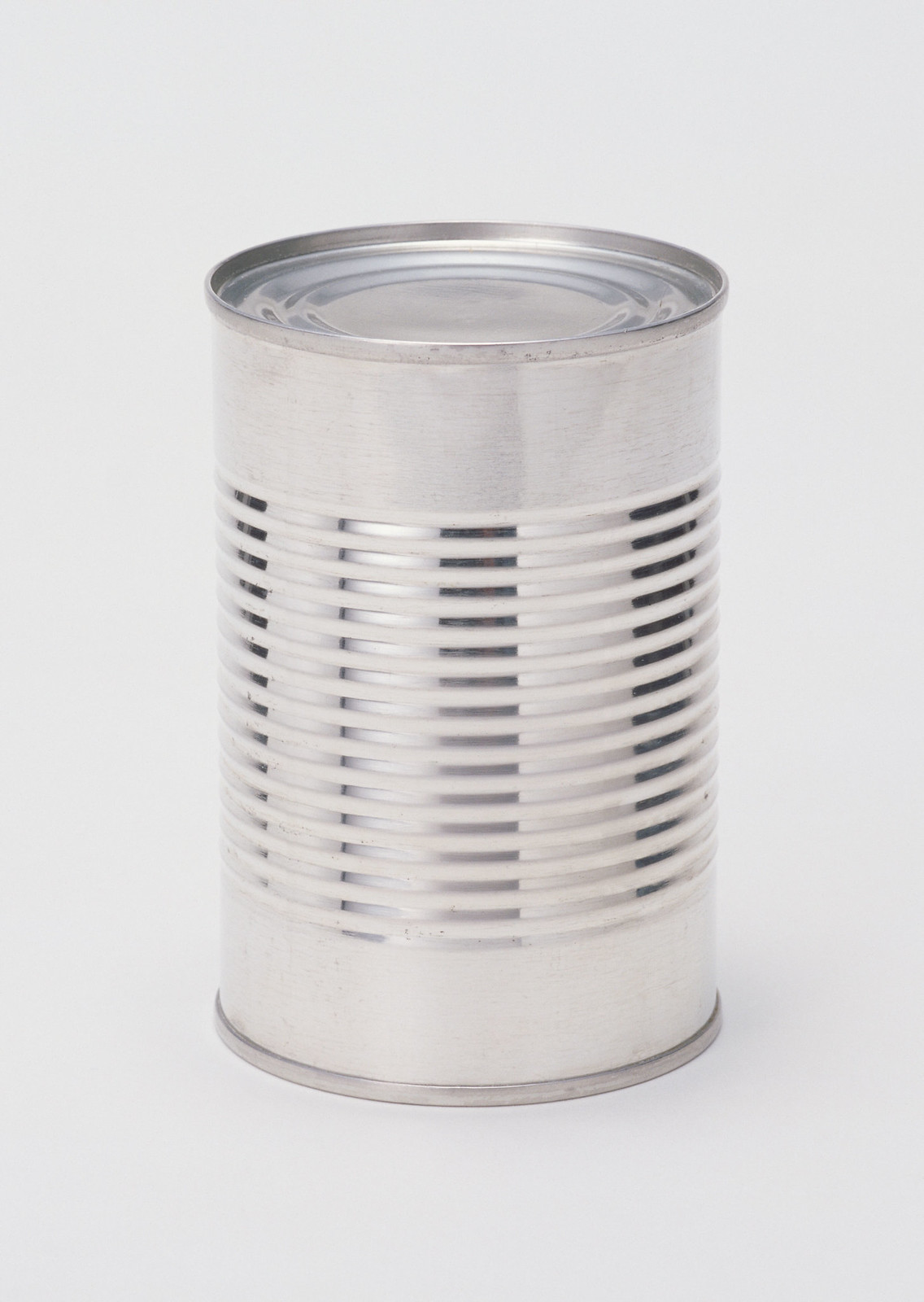This photograph features a standard 13-14 ounce tin can positioned centrally against a solid white background. The can is unlabeled, showcasing its stainless steel exterior. The body of the can has distinctive vertical ridges or stripes that create the appearance of small holes, offering a textured, almost grid-like design. At the top, a shiny silver lid reflects light, making the silver elements more pronounced. The can also has a silver band at the bottom, contributing to its reflective, metallic sheen. The entire surface of the can glistens under the light, enhancing its sleek, industrial look.